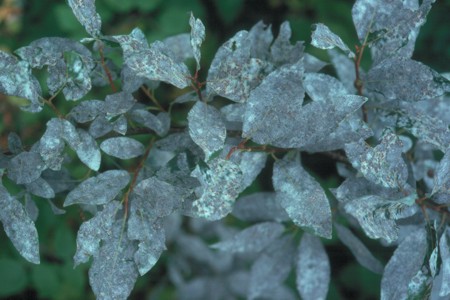The photograph, taken in landscape mode, presents a close-up view of a plant showcasing delicate, silver-blue to teal leaves, which feature intricate patterns and grooves, almost resembling a worn fabric or crystallized texture. The leaves have various shades of blue, including silver light blue and darker tones, combined with white speckles, creating a strikingly detailed and almost unreal appearance. The thin, red-brown stems adding contrast to the scene. The background is a blurred mix of green foliage, adding depth and emphasizing the main subject, with slight hints of orange in the top left corner. The focus remains sharply on the fragile, patterned leaves, lending them a three-dimensional quality against the softened backdrop.